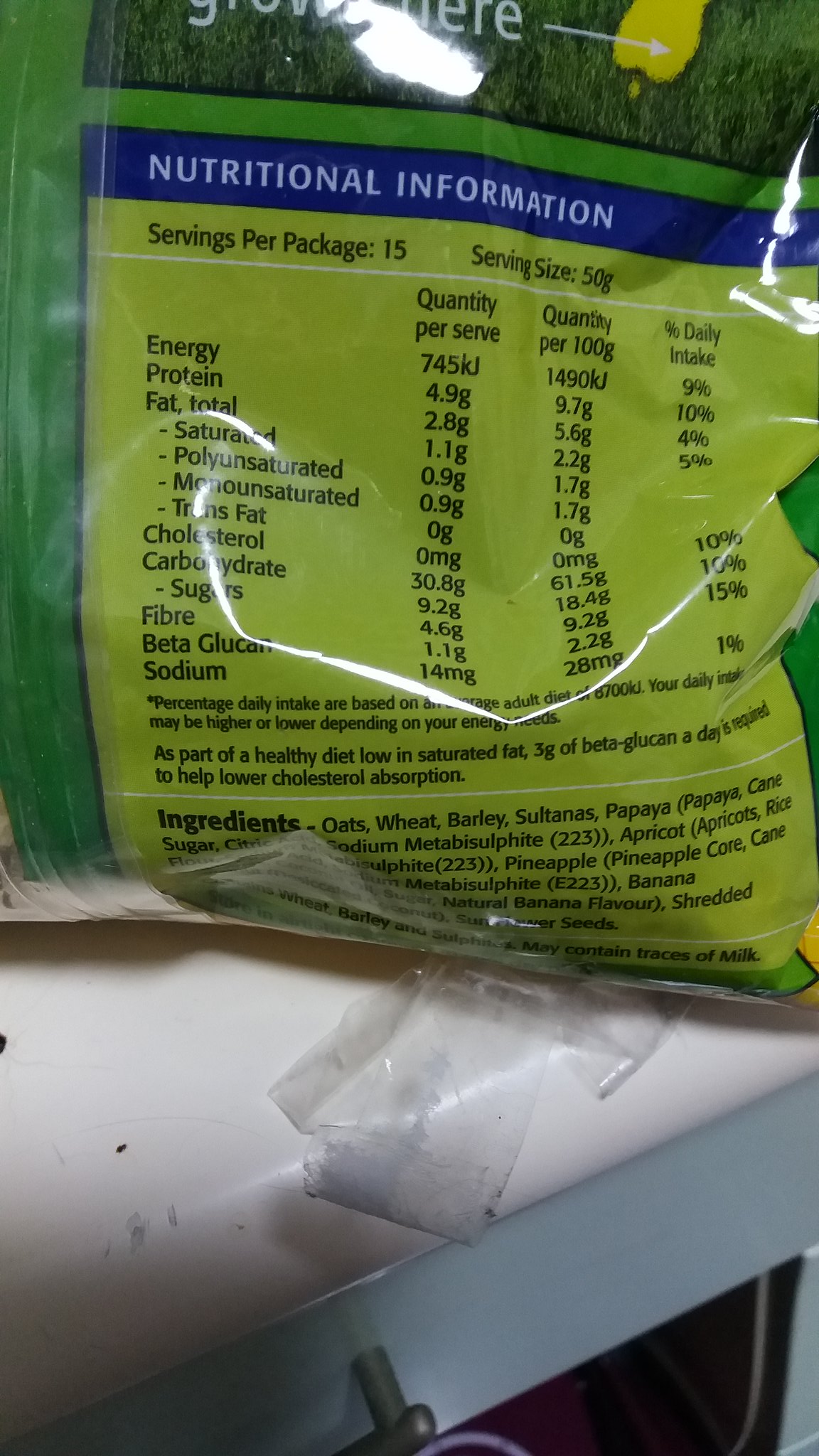A green food product package is displayed on a white countertop with a hint of a light green base peeking in from the edge of the image. The package features a detailed nutritional information section prominently displayed on a blue strip, labeled "Nutritional Information" in white text. Below this, a yellowish-green box with black print provides extensive details about the nutritional content of the product. The label specifies that each package contains 15 servings with a serving size of 50 grams. 

The nutritional information is organized into three columns: quantity per serving, quantity per 100 grams, and percentage of daily intake. The listed categories include energy, protein, total fat, saturated fat, polyunsaturated fat, monounsaturated fat, trans fat, cholesterol, carbohydrates, sugar, fiber, beta-glucan, and sodium. A note at the bottom explains that the percent daily intake values are based on an average adult diet of 8,700 kJ, warning that individual daily needs may vary. Additionally, it highlights the health benefits of consuming 3 grams of beta-glucan daily to help lower cholesterol absorption. Each nutritional element has corresponding totals neatly itemized.